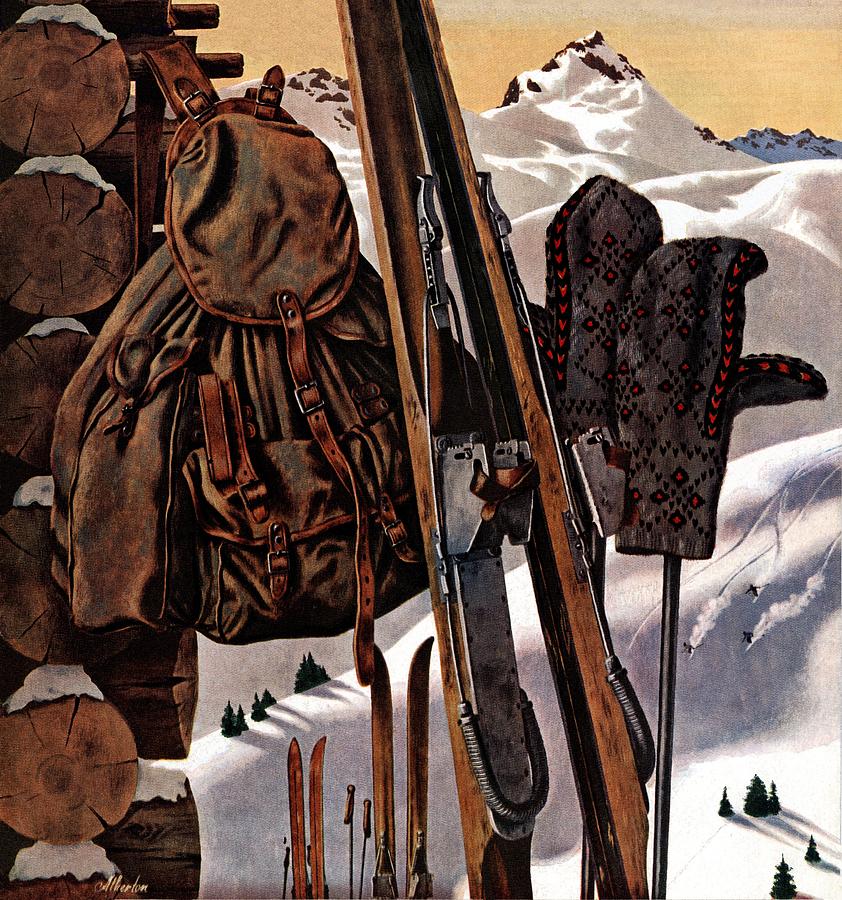This detailed drawing presents a captivating view from a log cabin situated high up in the mountains. The left side of the illustration showcases the sturdy, rustic logs of the cabin. Prominently displayed against the structure is an old-fashioned, weather-beaten leather backpack and a pair of brown skis, lying at rest with ski poles sticking upright in the snow. Draped over the ski poles are gray mittens adorned with red heart designs, adding a touch of warmth and homeliness to the scene.

In the middle ground, several skiers – approximately four – can be seen gracefully descending a snowy slope, kicking up a trail of powder as they race down. The snowy landscape is dotted with resilient green pine trees, their dark hues contrasting sharply with the surrounding white blanket of snow.

Beyond the skiers, the background reveals an awe-inspiring array of towering mountain peaks, each one more imposing than the last, and all glistening under a pristine blanket of snow. Enhancing the dramatic scenery further is an orange-tinged sky, casting a warm glow over the cold, wintry landscape.